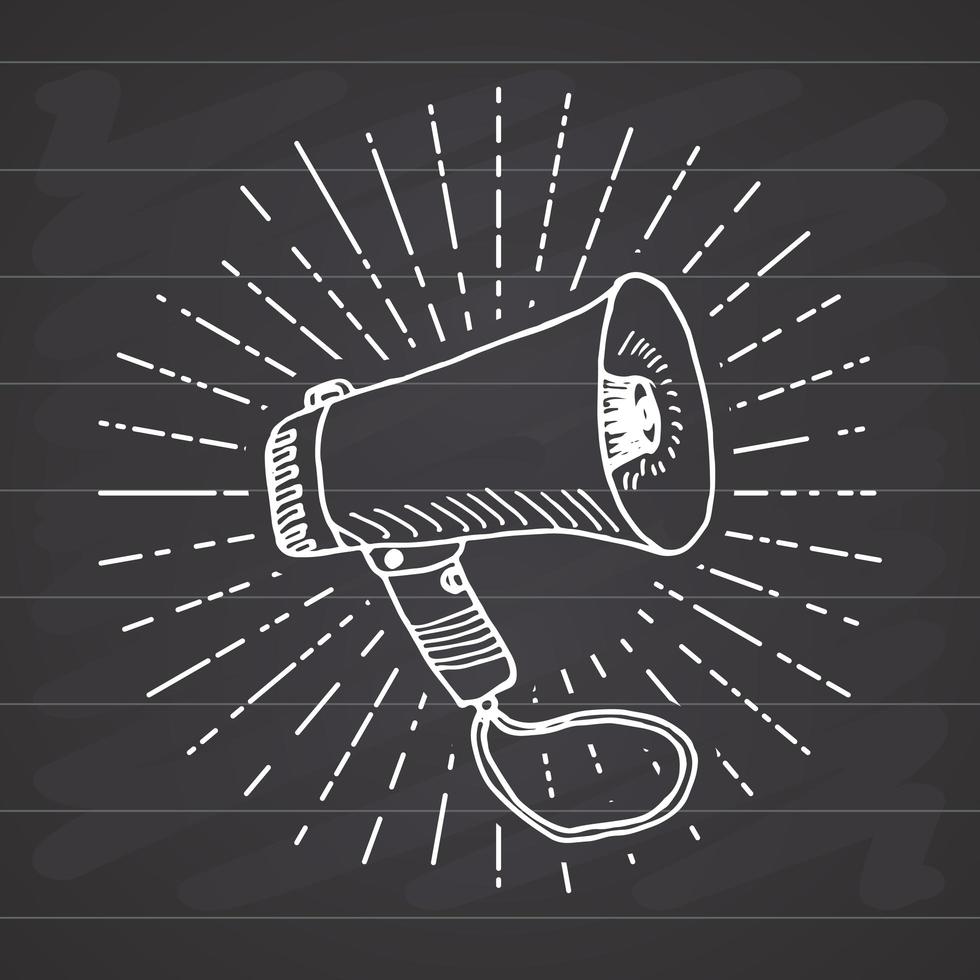The image is a detailed drawing of a megaphone centered on a black square background, which features nine thin, equidistant white horizontal lines giving the appearance of planks of dark wood. The megaphone, outlined intricately in white, points to the right and includes fine details such as a string loop at the bottom of the handle, possibly for carrying, and buttons and knobs on the handle and upper part. The body of the megaphone shows areas of shading with dashed lines to indicate depth. Surrounding the megaphone are broken, radiating white lines creating a sunbeam effect, visually emphasizing the sound emanating from it.